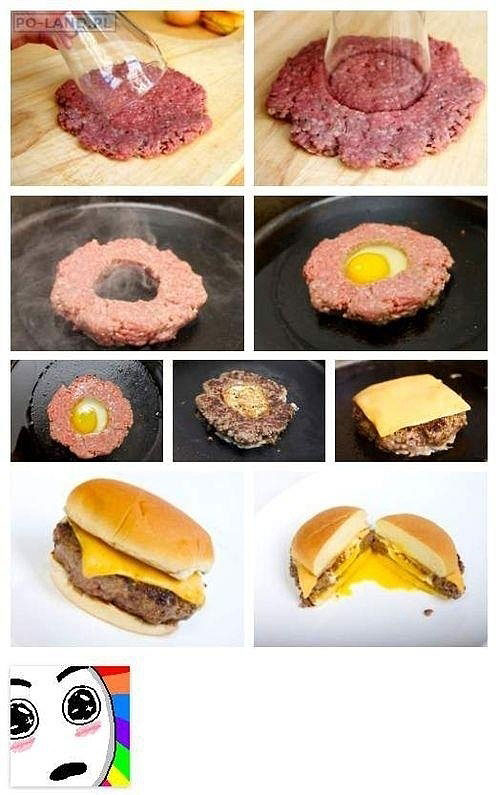A step-by-step tutorial on making a cheeseburger with a fried egg center is depicted in this series of images. 

1. The process begins with slightly smashing a hamburger patty.
2. Using a cup, the chef creates a hole in the center of the ground beef.
3. The raw hamburger meat is then placed in a hot pan, with the center portion removed, allowing it to cook.
4. An egg is cracked and added into the middle of the patty while it continues to cook.
5. The patty and egg are shown cooking together, with visible oil in the pan. The meat is transitioning from its raw pink hue to a more cooked state.
6. The burger patty with the egg in the center is flipped, revealing that the egg has mostly set, with a firm white and brown exterior, while some yolk remains visible.
7. A slice of American cheese is placed over the browned burger patty and egg.
8. The cheeseburger assembly is completed with a typical, untoasted hamburger bun.
9. When the burger is cut in half, the runny egg yolk is visible, oozing out.
10. The final image humorously illustrates the reaction to the culinary creation, featuring a cartoon face with sparkling eyes and a rainbow of colors (red, blue, orange, purple, green, yellow, pink) signifying astonishment and delight.